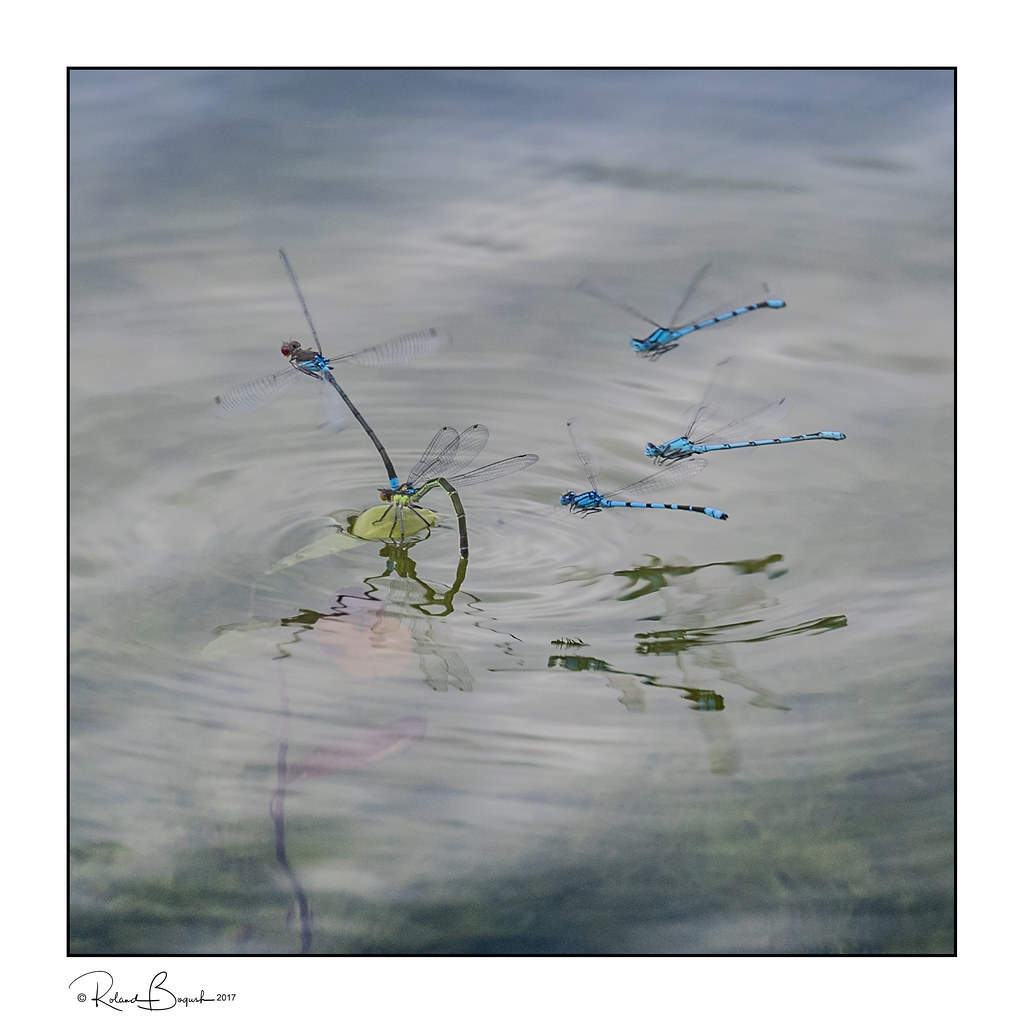This captivating close-up image, possibly a painting, showcases the serene surface of clear, shallow water—likely a pond or river. A cluster of five strikingly bright turquoise blue dragonflies dominates the scene. Four dragonflies are in flight, their horizontal orientation creating small ripples as they hover towards a central green leaf emerging from the water's surface. The fifth dragonfly perches gracefully on this leaf, its delicate body contrasting against the vibrant green. Reflections hint at shadows beneath the water, revealing some submerged vegetation, possibly grass. The water's transparency allows glimpses of the plants below, enhancing the image's tranquil and detailed natural beauty.